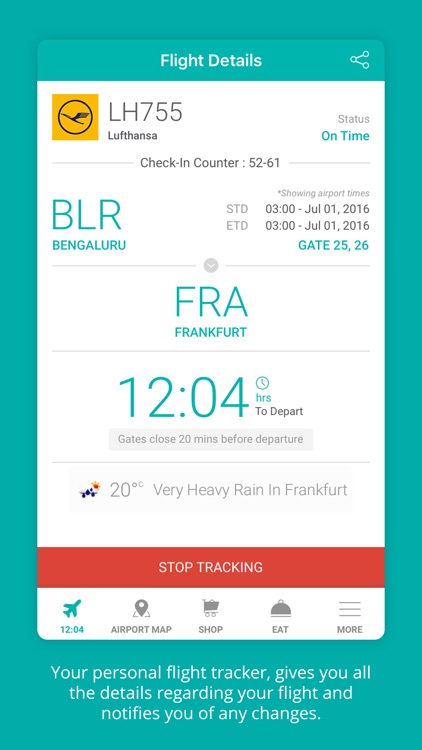Flight Tracker Details for LH 755 from Bengaluru to Frankfurt

This image displays a comprehensive flight tracker for Lufthansa flight LH 755, departing from Bengaluru (BLR) to Frankfurt (FRA). The main details are highlighted in various colors and sections:

- **White Text**: "LA 755 Lufthansa"
- **Yellow Square**: "Check-in counter 52 to 601"
- **Status**: "On time"
- **Black Text**: "STD: 03-July-1st-2016" and "ETD: 0300-July-01, 2016"
- **Blue Text**: "Gate: 25/26"
- **Gray-Blue Text**: "FRA Frankfurt"
- **Additional Information**: "12:04 hours to depart, gates close 20 minutes before departure"
- **Weather Condition**: "20°C with very heavy rain in Frankfurt"
- **Red Bar**: "Stop tracking"
- **Additional Features**: A blue plane icon, and options for an airport map, shopping, eating, and more
- **Footer Note**: "Your personal flight tracker gives you all the details regarding your flight and notifies you of any changes."

This organized flight tracker allows passengers to get real-time updates and detailed information about their flight, ensuring a smooth travel experience.